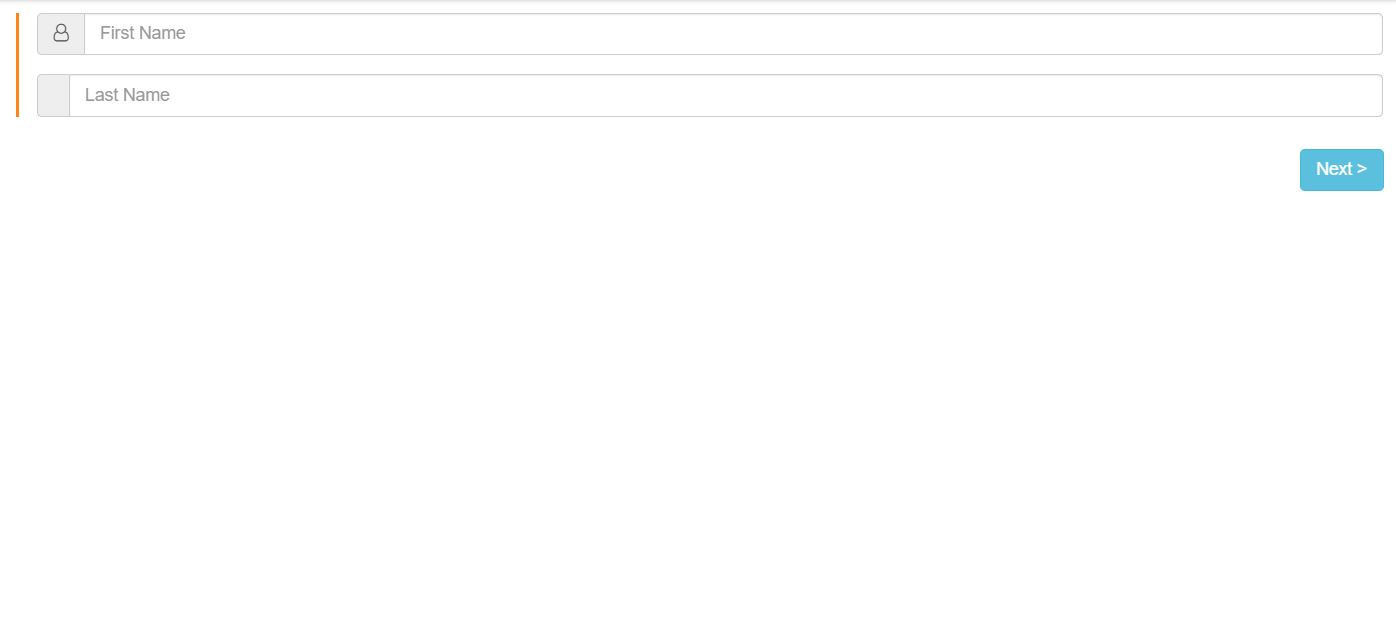The screenshot features a minimalist design with a predominately white background. At the top, a thin, light gray line stretches horizontally across the screen, creating a subtle separation. Positioned vertically on the right is a short, orange line that draws the eye to the main interactive elements of the image: two input fields for entering a user's first and last name.

The first name input box is distinguished by a light gray border and features an icon of a person's silhouette on a small, light gray square to the left. The placeholder text inside this box reads "First Name" in light gray, subtly prompting the user for their input. Additional spacing separates this from the second input box below, which bears similar features. It also includes a light gray icon box followed by the placeholder text "Last Name."

In the bottom right corner, a small, light blue rectangle button with white text labeled "Next" indicates the next step in the process. The overall design is clean and user-friendly, focused on simplicity and ease of navigation.